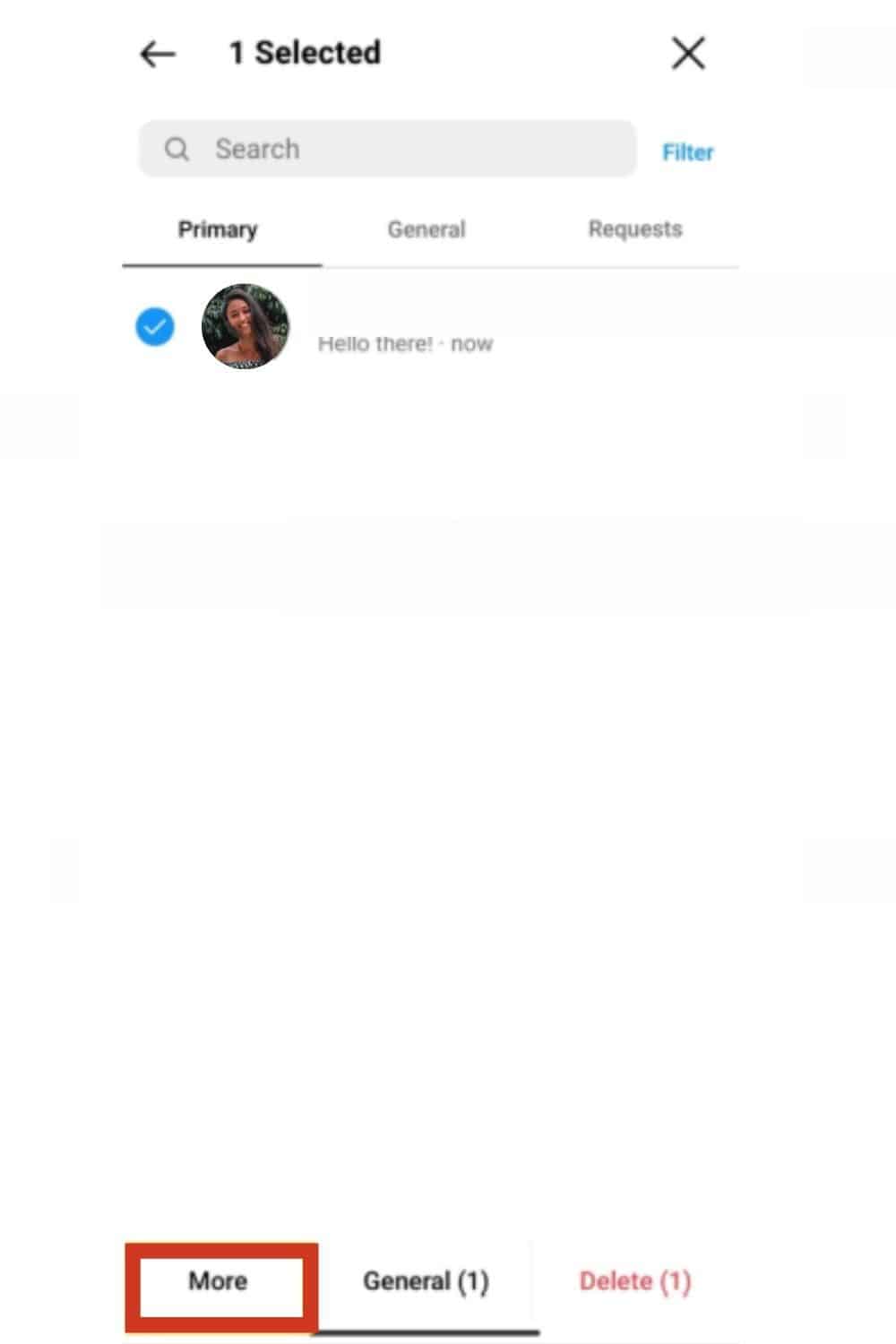This is a detailed screenshot of a cell phone interface, primarily featuring a white background. In the top left corner, there's a left-facing arrow indicating navigation to a previous menu, adjacent to the text "1 selected" in bold black font. On the far right, an 'X' icon is present for closing the screen. Immediately below is a light gray search bar, marked by a magnifying glass icon followed by the word "Search." To the right, the term "Filter" in blue suggests an option to modify settings.

The interface offers three tabs below the search bar: "Primary," "General," and "Requests." The "Primary" tab is selected, highlighted in black with an underline. Under this section, a circular profile picture of a young woman is displayed. To the left of her picture is a small blue circle containing a white tick. Adjacent to her image, the message "hello there" is displayed with a timestamp of "now."

At the bottom of the screen, in the lower left corner, the word "More" appears, encased in a bold red rectangular outline. In the center, the word "General" is displayed with a number in brackets, indicated as "1." On the far right, another option, "Delete," is similarly annotated with the number "1" in brackets.